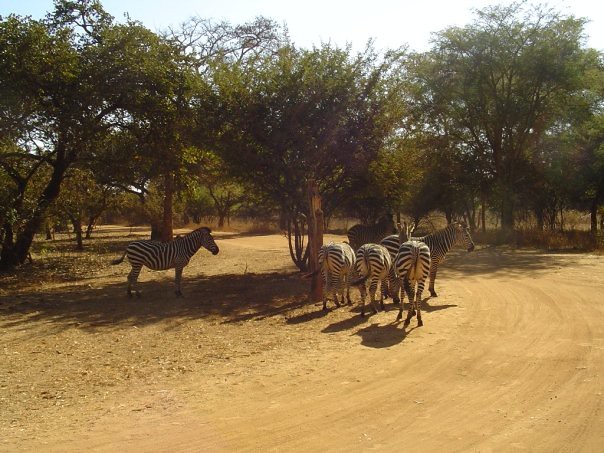This photograph captures a tranquil safari scene along a tan, sandy dirt road that curves from the right to the left and then disappears into the distance. The road features a well-worn, pebbly path on the left side, emphasizing its frequent use. Prominently, a group of six zebras with distinctive black and white stripes and equine-like physiques is seen inhabiting the area. On the right side, five zebras are mostly illuminated by sunlight, displaying their dark hooves, manes, muzzles, and tails. Three of them present their hindquarters to the viewer, while another faces right and slightly more in the background. On the left side, one zebra stands alone in the cool shade of a tree, facing right. Two large deciduous trees with green leaves at the foreground cast shadows over the dirt path. The background is lush with a tree line of similar deciduous greenery, providing a picturesque backdrop to the scene.